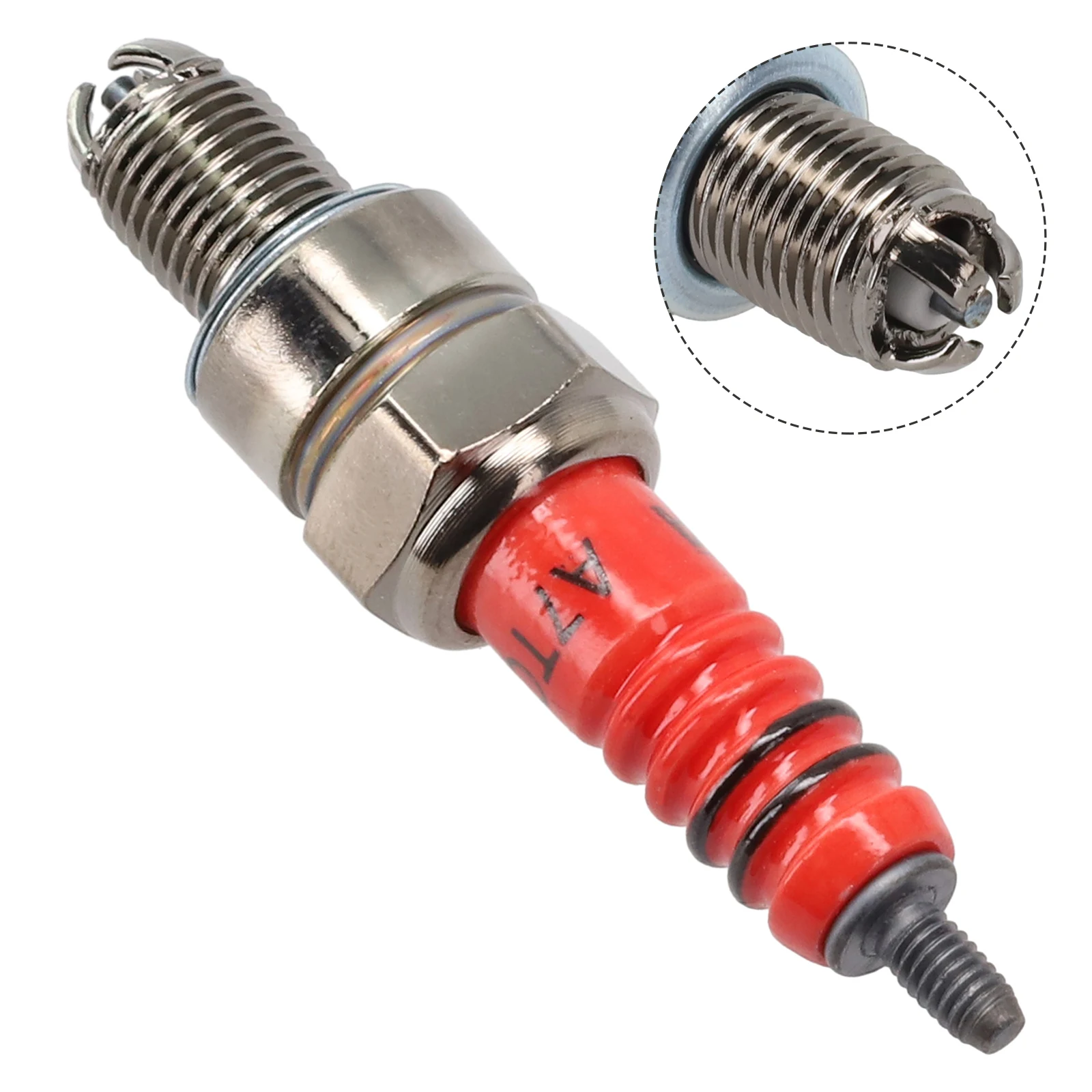This image displays a detailed view of a spark plug, predominantly featuring silver and red colors. The spark plug extends from the top right to the bottom left of the frame, against a nondescript background. The top portion sports a silver, spiral screw designed with approximately 10 notched lines descending from the top. Nestled in the middle is a red base marked "A7T," encircled by four distinct rings—the upper two rings are red, while the lower two are black. Attached to the base, at the bottom, is a standard-sized metal screw. Additionally, the top left corner of the image includes a close-up inset that highlights the top of the spark plug, showcasing a tri-pronged configuration, a coil-like design, and a white plastic interior with a cylindrical metal part protruding from it. This inset offers a clearer perspective on the connector type of the spark plug, aiding in identifying its compatibility.